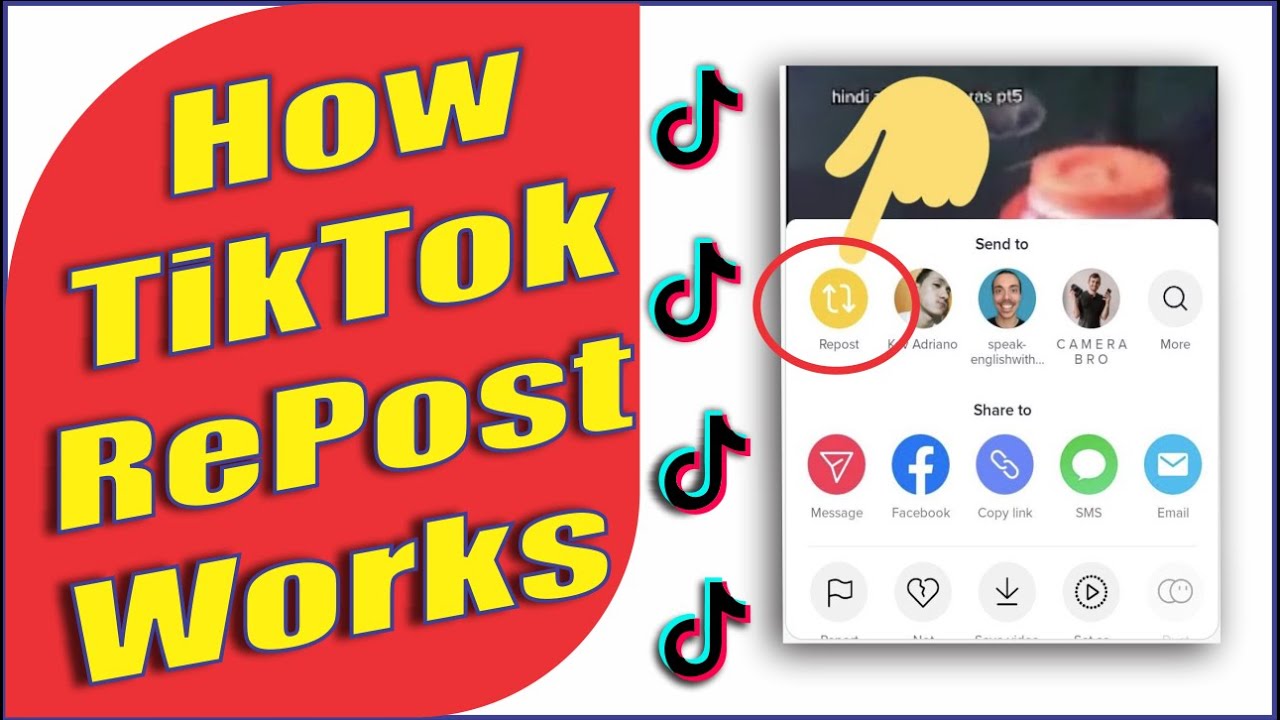**Detailed Caption:**

The image is a detailed YouTube video thumbnail, depicted in landscape mode with a prominent black border framing the entire scene. On the left side of the thumbnail, a red shape with bold yellow letters announces the topic: "How TikTok Repost Works." Adjacent to this are multiple vertical stacks of TikTok icons arranged in an orderly fashion.

Dominating the right side of the thumbnail is a screenshot of a smartphone interface. Notably, a post-production element included is a yellow hand with an extended index finger, emphasized by pointing at a specific icon on the interface labeled "Repost." The Repost icon is distinguished by a couple of arrows forming a circular motion.

This icon appears within a floating palette titled "Send To." Within this palette, the Repost option is clearly circled, highlighting its importance. Other sharing options visible on the palette include options to share with specific TikTok users like “Can Adriano speak English with…” and “Camera bro,” as well as the possibilities to share via message, Facebook, copy link, SMS, or email.

Below the smartphone interface, there are several additional icons: a flag icon, indicating a report or bookmark feature; a broken heart for dislikes or broken content; an arrow pointing downward at a line that may denote download or save; a dotted circle with a play button which likely suggests a replay option; and, lastly, two circles, one of which has eyes, possibly representing the Viewer or Watcher function.

This composition effectively guides viewers on what to expect from the video, offering a comprehensive breakdown of TikTok's repost functionality and various sharing methodologies within the app.